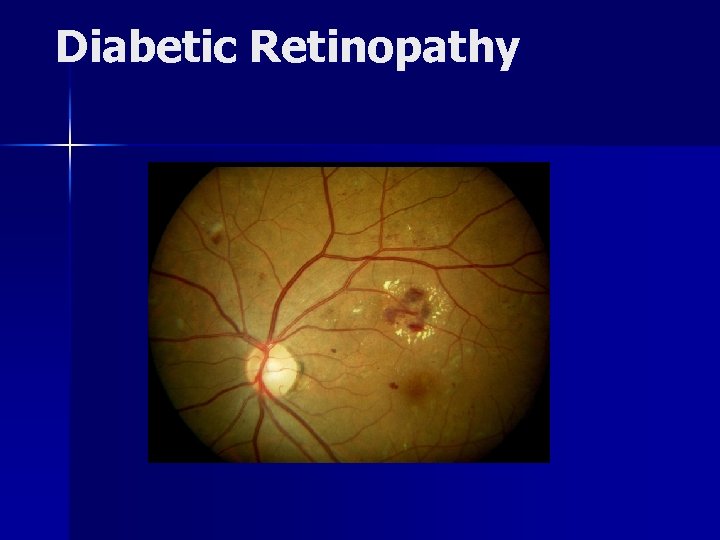The image, titled "Diabetic Retinopathy," features white sans-serif font at the top against a predominantly blue background, often seen in doctor’s offices or hospitals. A distinctive white and light blue cross extends from the top-left corner and stretches across the length and width of the poster, dividing the blue areas. Centrally positioned is a circular depiction resembling an eyeball or a close-up view under a microscope. The eye-like image has a dark gold or yellow hue, populated with a network of red veins, some thick and others thin. There are deep red indentations or lesions, especially prominent in the upper right area of a bright white spot near the center. The red veins appear bloody, converging towards this white, light-reflecting region, suggesting focused illumination. The detailed visual presents a clear medical illustration of diabetic retinopathy, highlighting the severity of blood vessel damage caused by the condition.